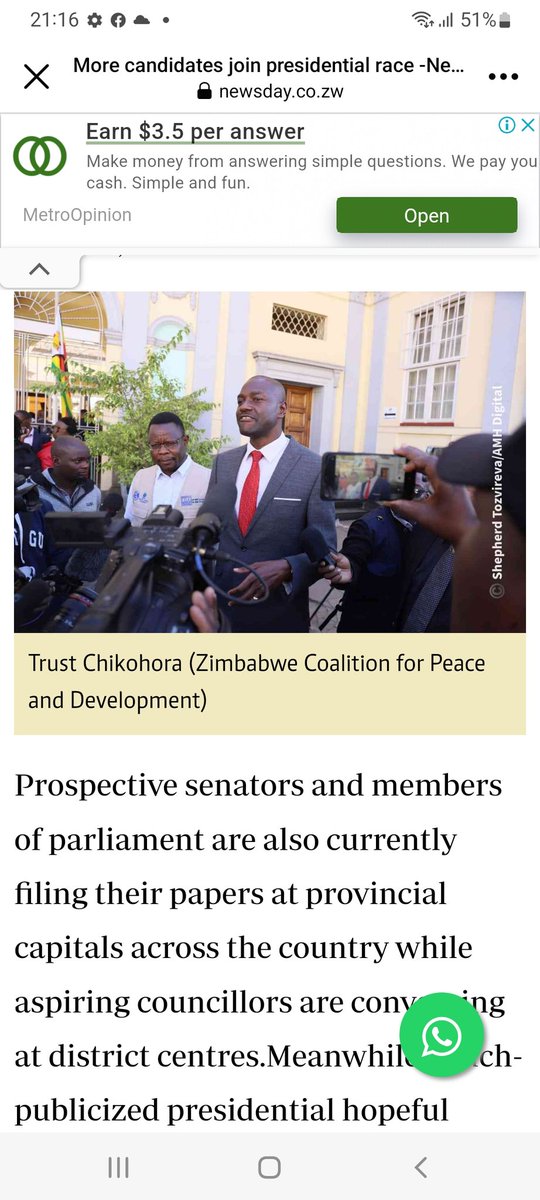The screenshot from a mobile phone showcases various elements against a white background at the top and features black font. At the very top, the time is displayed as 21:16, accompanied by several icons: a settings gear icon, a Facebook icon, a cloud icon, and Wi-Fi and mobile signal icons showing a 51% battery level. Below this, there is a large black "X" with the text "More candidates join presidential race - Ne..." to its right.

Further down, the screen shows the logo of "NewsDay" with the URL "newsday.co.zw." Underneath this, there is a vibrant banner ad reading, "Earn $3.5 per answer. Make money from answering simple questions. We pay you cash. Simple and fun. Metro Opinion."

The focal point of the screenshot is an image of a prospective senator for the Zimbabwe coalition, named Trust Chikora. He is depicted as a Black man dressed formally in a gray suit, a red tie, and a white shirt. Trust Chikora stands confidently at a podium, with reporters and their cameras focused on him. In the background, a pleasant blue house is visible, lending a sense of location to the setting.